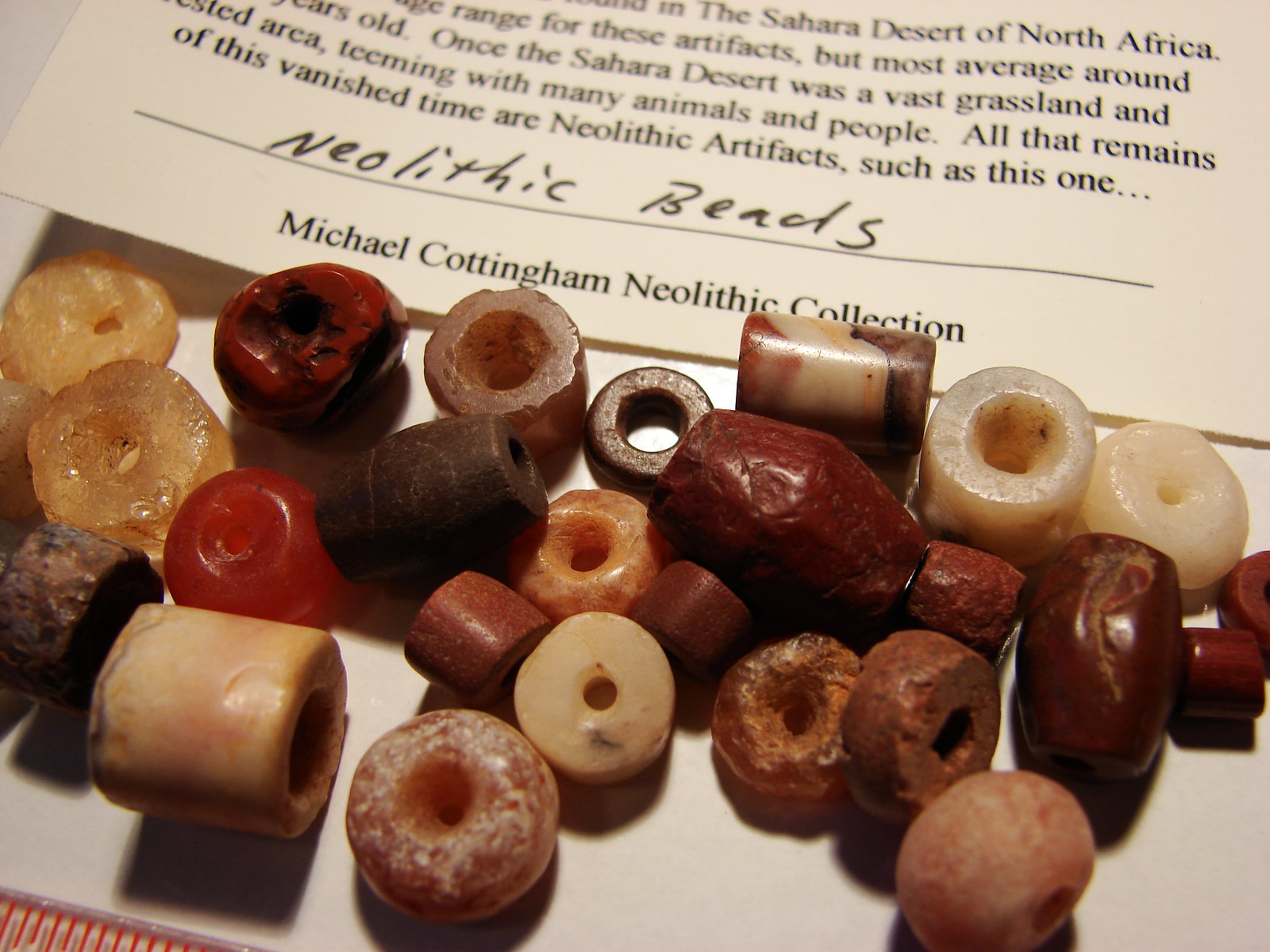This detailed image likely taken in a museum showcases an assortment of Neolithic beads scattered across a white surface at the bottom of the frame. The beads vary in size, shape, and color, including white, black, brown, orange, yellow, and maroon. Some beads are donut-shaped with large holes, while others are tube-shaped with smaller apertures. The upper portion of the image features the lower half of a sheet of paper with printed and handwritten text. The paper includes a black line across it, below which is the text "Neolithic beads" and "Michael Cottingham Neolithic Collection." Above this line, the partially visible text describes the Sahara Desert's transformation from a grassland teeming with life to its current arid state and notes the presence of artifacts from the Neolithic era. The setting appears to be indoors, adding to the impression of a curated display, possibly within a museum exhibit.